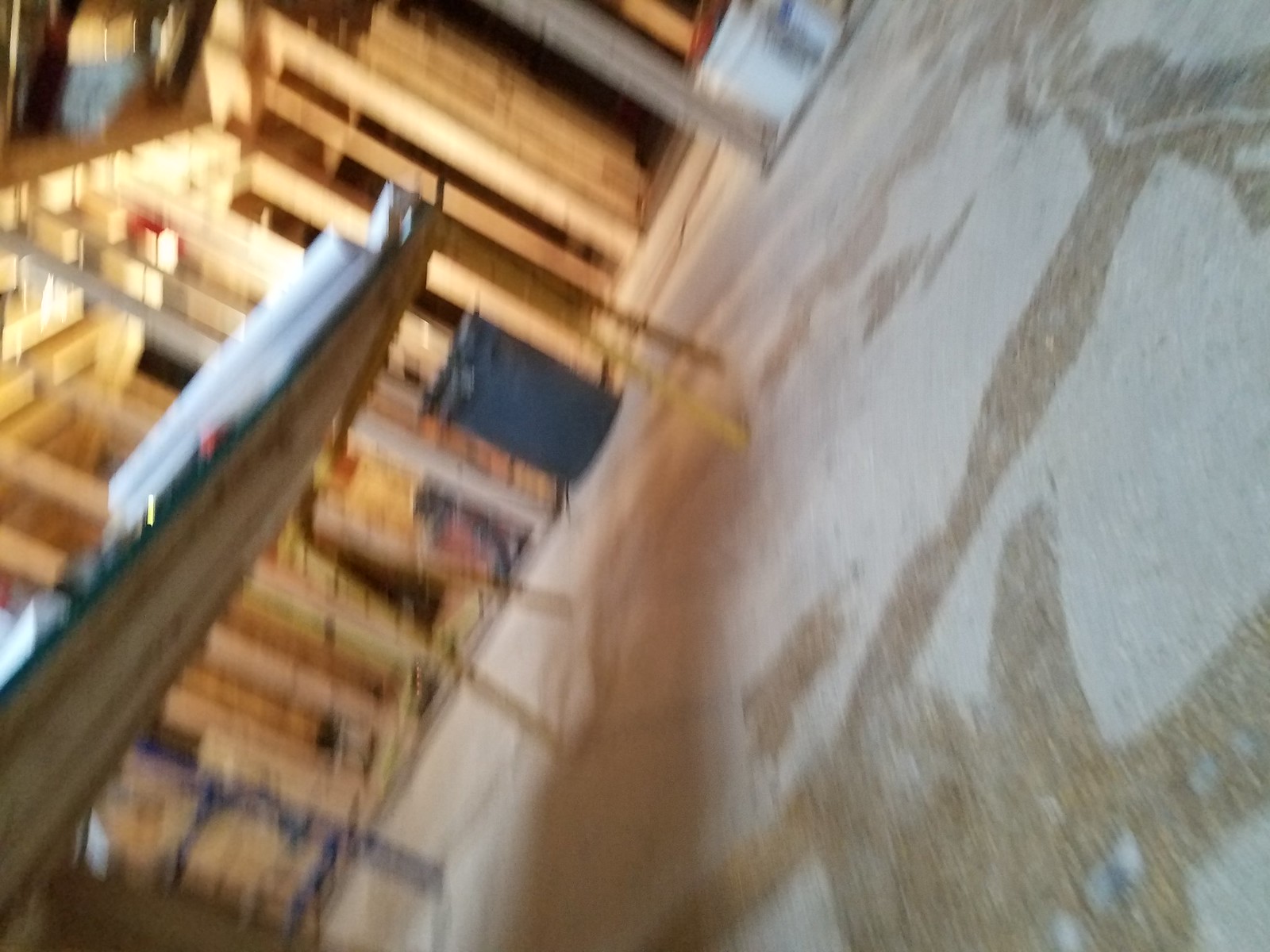This vibrant color photograph captures the interior of a house under construction. Positioned likely with the camera lying sideways on the concrete floor, the image is oriented such that the floor appears on the right side of the frame. To the left, a makeshift work area is set up with a table, laden with tools and building materials. The skeletal framework of the house is prominently featured, showcasing numerous four-by-fours and two-by-fours that define the structure. In the background, a gray trash can is visible, adding to the authentic, in-progress atmosphere of the site. The concrete floor is marked with glue filling in the cracks, highlighting ongoing efforts to secure and stabilize the foundation. The photo encapsulates the raw, industrious essence of home construction.